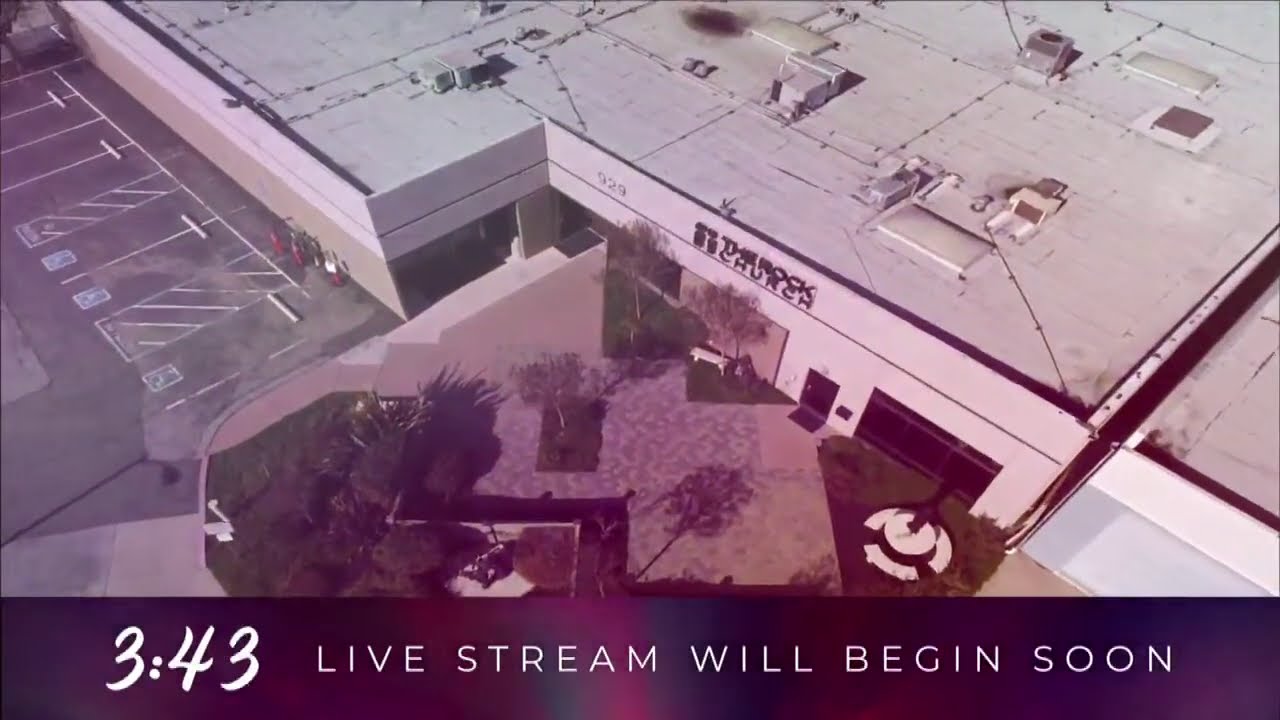This image is an overhead drone shot, showcasing a large, one-story building with an extensive floor plan, identifiable as The Rock Church with the building number 929 visible on the wall. The flat white roof is dotted with air conditioning units, piping, and plumbing. In front of the building, there's a plaza area featuring trees, bushes, a small circular picnic table, and a couple of benches, all set against tan and brown ground hues. Adjacent to the plaza lies an empty parking lot with clearly marked spaces, including handicapped spots highlighted in blue and white. The entire scene has a sepia-toned appearance, lending it an aged, cinematic feel. At the bottom of the image, there is a purple banner displaying the text "343 LIVE STREAM WILL BEGIN SOON" in white capital letters, with "343" being more prominent. This overlay suggests the image is part of a video feed, likely a YouTube livestream countdown for the church.